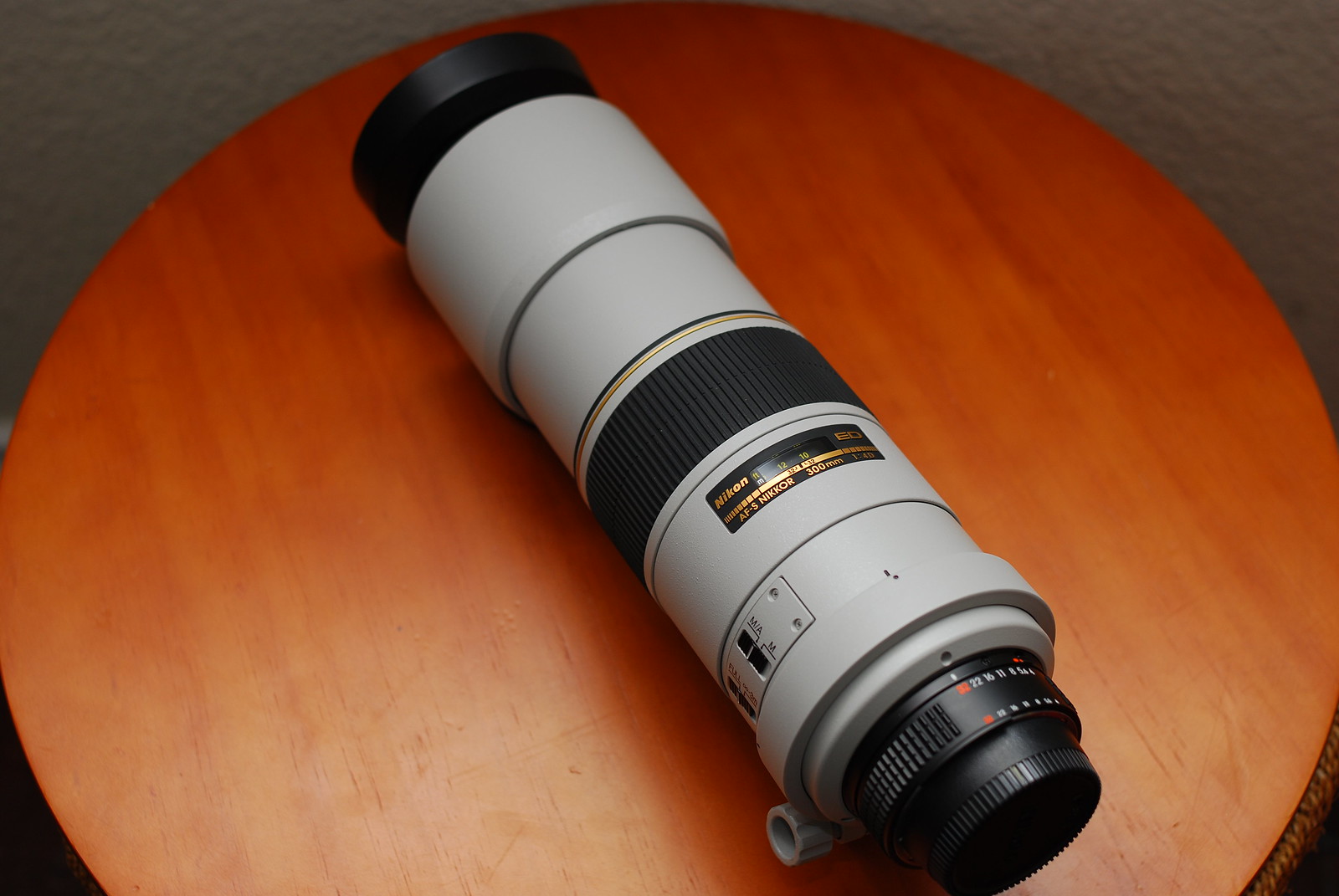A large, professional-grade camera lens is prominently displayed on a round, shiny, brown tabletop, likely made of maple wood. The lens stretches diagonally from the upper middle left to the lower middle right of the table, which is situated on a gray rug. The lens itself features black ends and a black band around its middle, with a predominantly off-white or gray body. Notable details include a black cap on one end, black dials on the other, and a small black window or tag with gold writing. The tabletop has a very polished and clean appearance, enhancing the overall presentation of the camera lens.